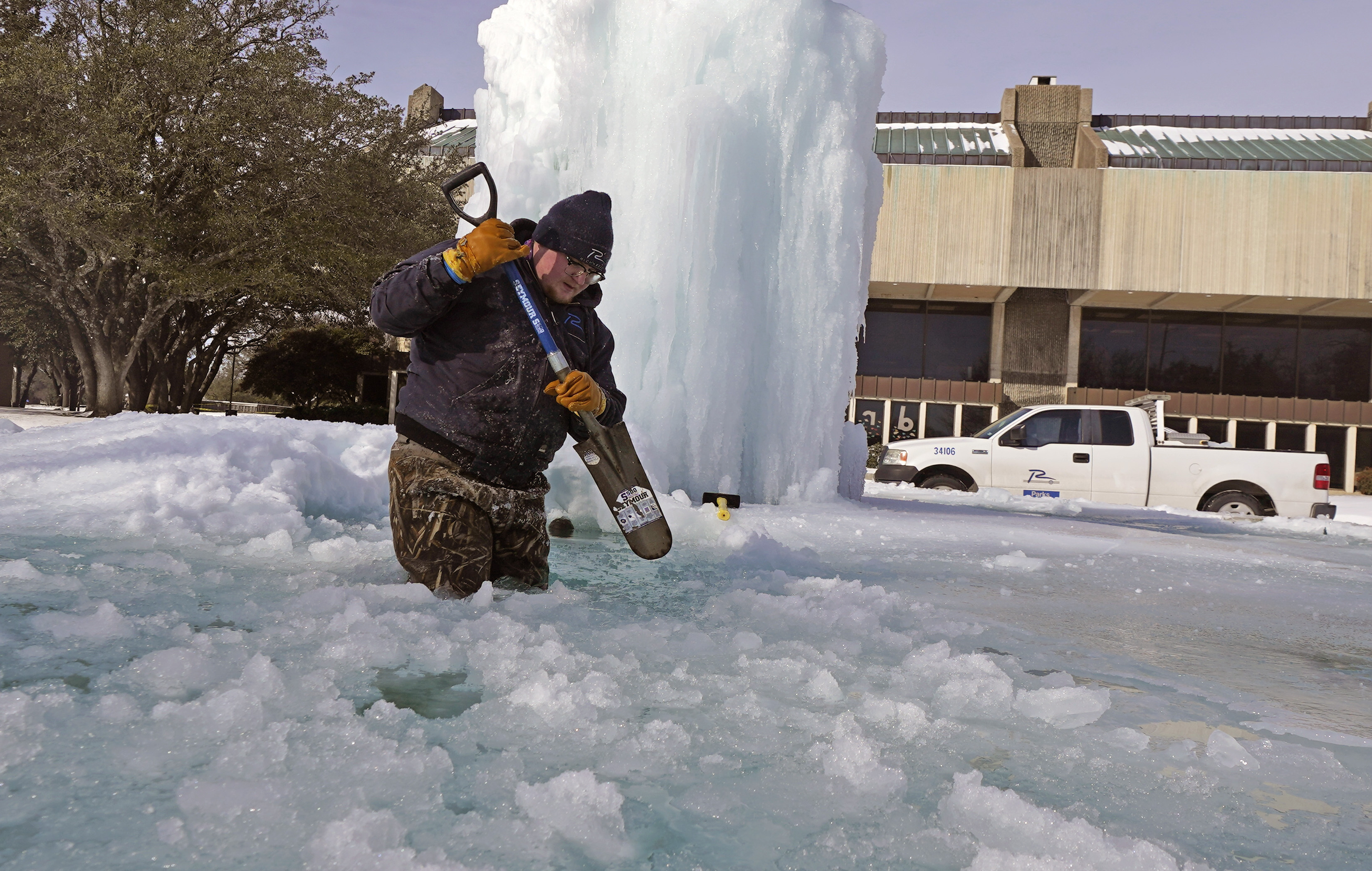In this photograph taken on a wintry day, a young, heavyset white man is captured as he stands thigh-deep in a frozen, waterlogged area, seemingly working to break up the ice. He is dressed in a navy blue winter jacket, a matching ski cap, brownish-green camouflage pants, and tan-colored work gloves. He holds a shovel, poised to dig into the icy surface. Behind him stands a large, monolithic ice sculpture, formed from a frozen fountain that has created a dramatic display of fused icicles. The setting includes a cement building with smoky glass panes and the number 76 prominently displayed on its façade. A white work truck is parked in front of this building, which has a little snow on its green metal roof. To the man's left, a grove of trees retains some green leaves, adding a touch of color to the otherwise wintry scene.